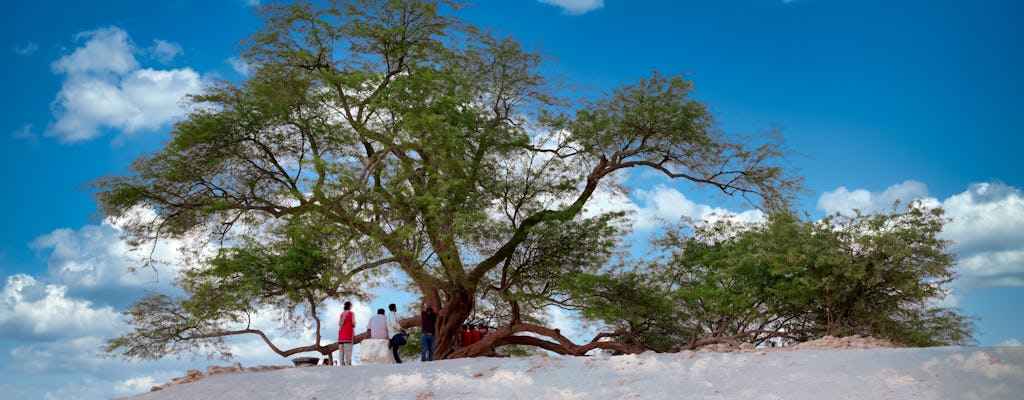The image depicts a picturesque outdoor setting featuring a large tree with a brown trunk and lush green foliage, prominently set against a bright blue sky dotted with puffy white clouds. At the base of the tree stand three individuals – one woman and two men – all facing into the distance. The woman, dressed in a bright pink or red sleeveless top and white pants, carries a shoulder bag. One of the men is adorned in a traditional Indian kurta, possibly in a purple shade, while the other is in dark pants paired with a light-colored shirt. They stand on a gray or sandy ground.

To the right of the large tree is a smaller, bushy green plant, which complements the vibrant greenery of the scene. Additionally, several children in red shirts can be seen sitting on one of the tree's branches, adding a playful element to the serene landscape. Among the people beneath the tree, there is a small, round table positioned near the woman.

In the background, various details such as short, brown rocks and a white hill can be gleaned, adding texture to the landscape. The overall composition captures the tranquility and natural beauty of the scene, with the expansive sky enhancing the sense of openness and peace.